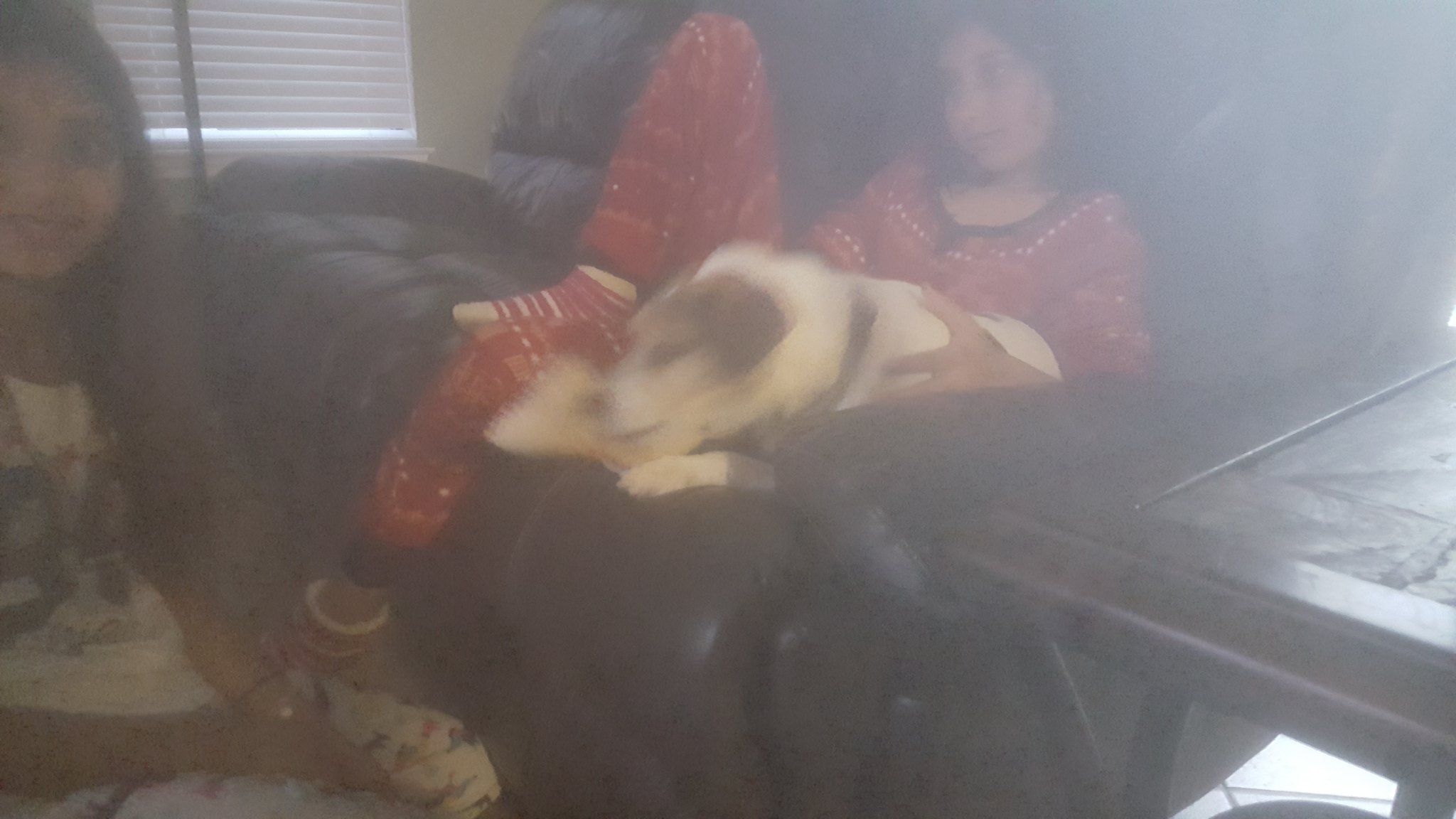In what appears to be a living room, a blurry photograph captures a youthful and cozy moment. On the left side of the image is a young individual with long brown hair, clad in a white shirt and matching white pants, both adorned with a distinctive design. The central focus of the photograph is a black leather couch, occupied by another young person who exudes a comfortable and relaxed demeanor. She is wearing red and white patterned pajamas, her dark hair complementing her tan complexion. Beside her on the couch is a white and brown dog, adding a touch of warmth to the scene. To the right of the couch, a glimpse of a table corner is visible, hinting at the familiar, lived-in atmosphere of the room.